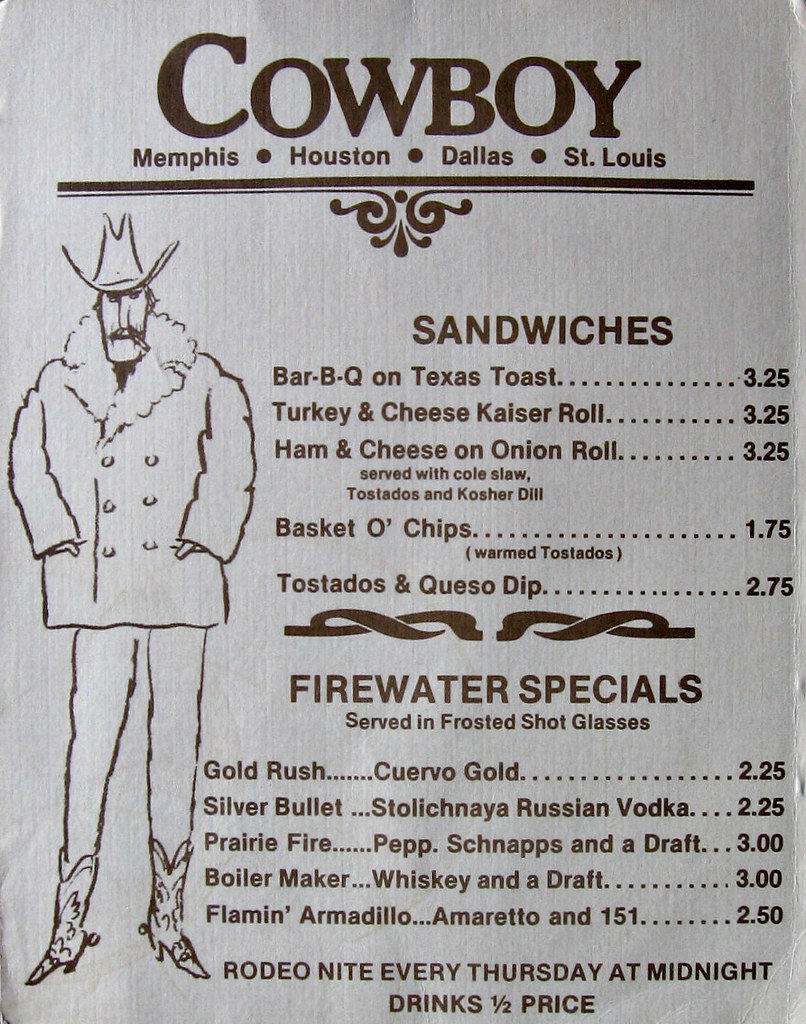The image depicts a detailed poster advertising a menu. The poster is predominantly white with all text written in brown ink, giving it a rustic feel. At the top, the word "Cowboy" is prominently featured. Below "Cowboy," there are the words "Memphis, Houston, Dallas, and St. Louis" listed, suggesting different menu items or themes related to these cities. A horizontal line separates this section from the rest of the content.

The menu itself includes several options: 
- Barbecue on Texas toast
- Turkey and cheese rolls
- Ham and cheese rolls

Each of these items is priced at $3.25.

Below the menu, there is a horizontal line with a unique KD design. The menu also highlights a "Fire Water Special," which is served in frosted shot glasses, with prices ranging from $2.25 to $3.00.

At the bottom of the poster, a promotional detail is included: "Rodeo Night every Thursday at midnight - drinks half price." 

On the left side of the poster, there is a detailed drawing of a cowboy. The cowboy is depicted wearing a cowboy hat, with a cigarette in his mouth, hands in his pockets, dressed in a jacket, and sporting cowboy boots. This illustration adds a visual element that enhances the Western theme of the poster.